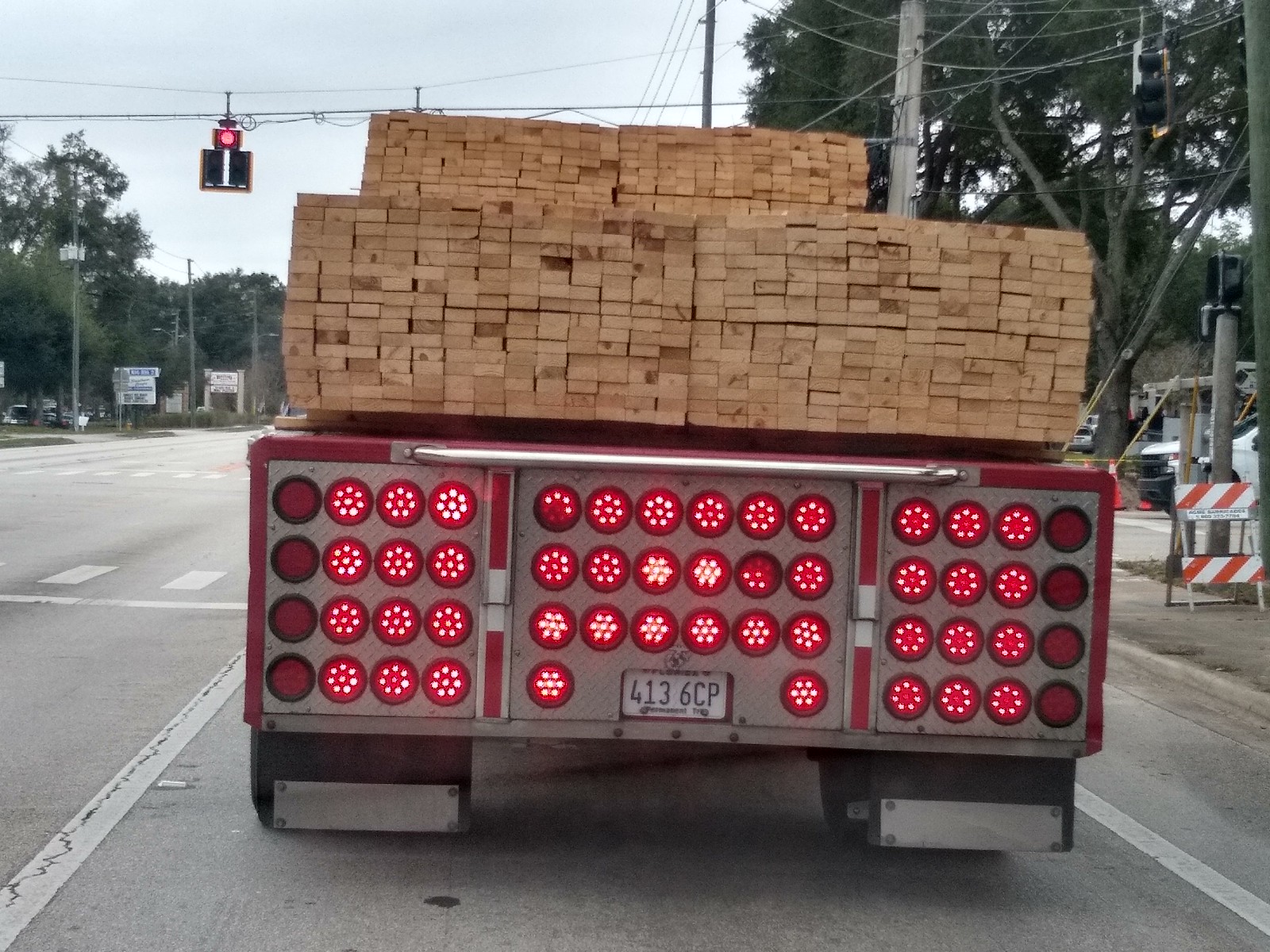This rectangular, horizontal color photograph captures the back end of a flatbed truck transporting numerous long, thin slats of brown wood. The flat pieces are stacked in organized blocks, appearing neatly wrapped around the bed of the truck. The truck itself is predominantly red, including its rear where multiple lights are arranged. Specifically, there are three distinct blocks of lights: one block of four rows of four lights on the left, one block of three rows of six lights in the middle, and another block of four rows of four lights on the right. Most lights are lit and glowing red, indicating the truck is stopped, likely at a stoplight. Notably, some lights in the left and right columns are not illuminated. The truck also features an American license plate bearing the number 4136CP. On the left side of the photo, a street lined with trees is visible, while the right side suggests ongoing roadwork. Additional details include a silver metal pole on the truck and white road markings, with one cracked line visible.